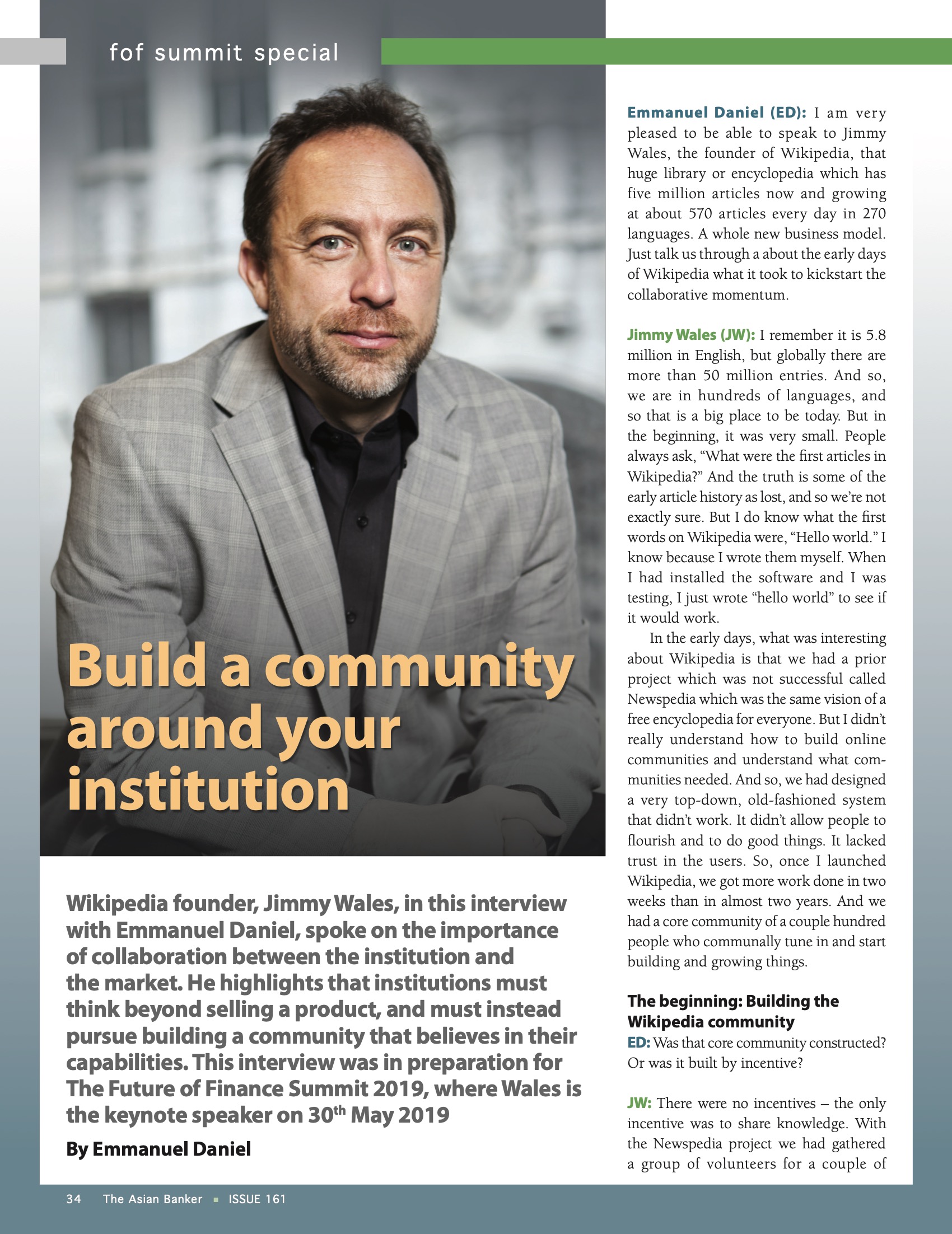Prominently displayed in this image, a screenshot from a magazine feature, is a photograph of Emmanuel Daniel. Dressed in a gray suit paired with a black shirt, Daniel sports a beard and a slightly receding hairline. Beneath his image, bold text declares, "Build a community around your institution."

The accompanying article features a discussion between Emmanuel Daniel and Wikipedia founder Jimmy Wales. Daniel and Wales emphasize the significance of fostering collaboration between institutions and the market. They argue that institutions must transcend mere product sales to focus on community building that inspires trust in their capabilities.

The interview was conducted in anticipation of the Future of Finance Summit 2019, where Wales was the keynote speaker on May 30, 2019. In the excerpt, Emmanuel Daniel expresses his pleasure in speaking with Jimmy Wales, noting Wikipedia's impressive scale with over 5 million articles and an addition rate of about 570 articles per day in 270 languages. Daniel prompts Wales to recount the early days of Wikipedia and the efforts required to generate the collaborative momentum that now defines the platform. The text captures their engaging conversation on business models and the evolution of collaborative digital platforms.